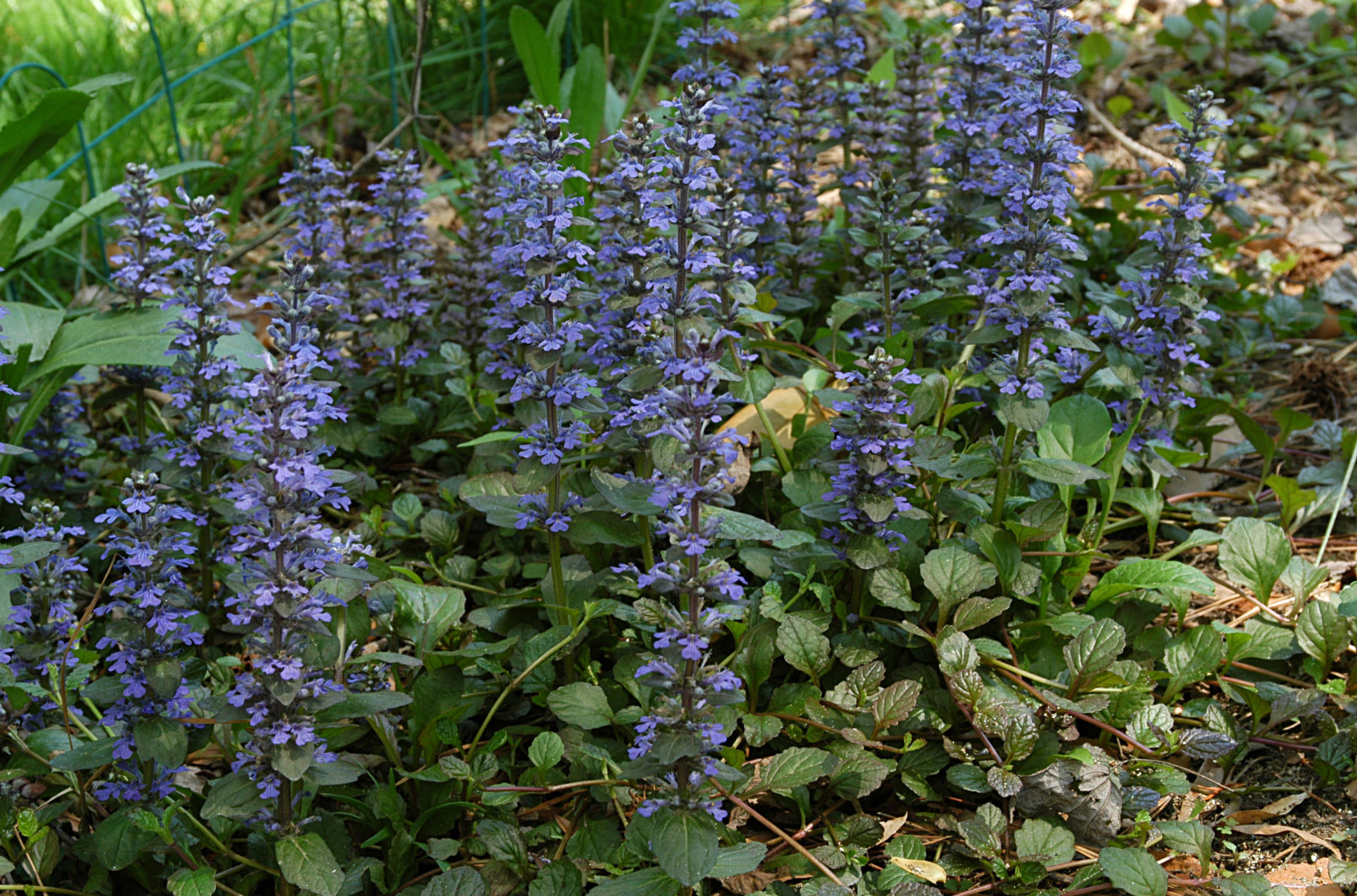This photograph captures a vibrant natural scene featuring approximately 25 tall, thin, long-stemmed wildflowers with clusters of delicate purple blossoms. These blossoms, which exhibit a striking bluish-purple hue, are scattered along the entire length of the stems, rising about 18 to 24 inches above the ground. At the base of these wildflowers, an array of green, round, oval-shaped leaves blankets the soil, with smaller weeds, blades of grass, and some dead leaves interspersed among them. The background reveals additional green foliage, creating a layered, textured effect within this outdoor garden setting. The image is taken during the daytime and emphasizes the vivid cluster of purple flowers, showcasing their intricate beauty and height contrasted against the lower green vegetation.